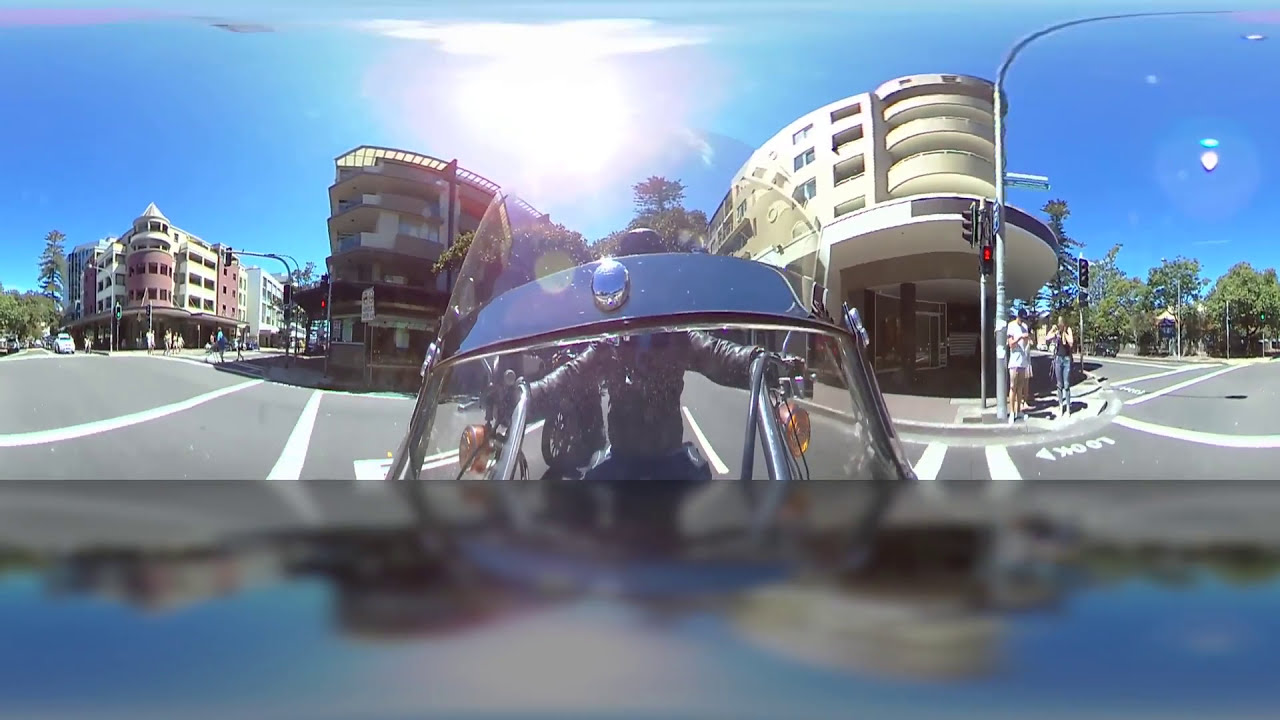The image captures a bright, sunny day with a clear blue sky, viewed from the perspective of a 360-degree camera mounted on a motorbike. Dominating the center foreground of the shot is the reflective, chrome-framed windshield of the bike, along with the chopper-style high handlebars and a visor showing reflections of the sun. The rider, wearing a black leather jacket and helmet, grips the handlebars firmly, both arms extended. There are small orange indicator lights on the bars.

In the background, the scene expands into a bustling urban intersection that forms a V-shape. On the left side, a cone-shaped building in the distance has rounded edges and is primarily white and light brown. The central building behind the rider is about six stories high, while to the right, a five-story, completely white rounded-edged building stands prominently. Traffic lights are visible in front of this white building, highlighting the busy crosswalks below. 

People can be seen standing at the crosswalks on both sides, waiting to cross the street. In front of the bike, near the bottom of the image, there's a metal bar and the edge of a glass shield, likely part of the motorbike. Text painted on the road reads "LOOK" with an arrow pointing left, guiding pedestrians.

The detailed scene reflects the urban environment's vibrant activity and the careful orchestration of vehicular and pedestrian movement within it.